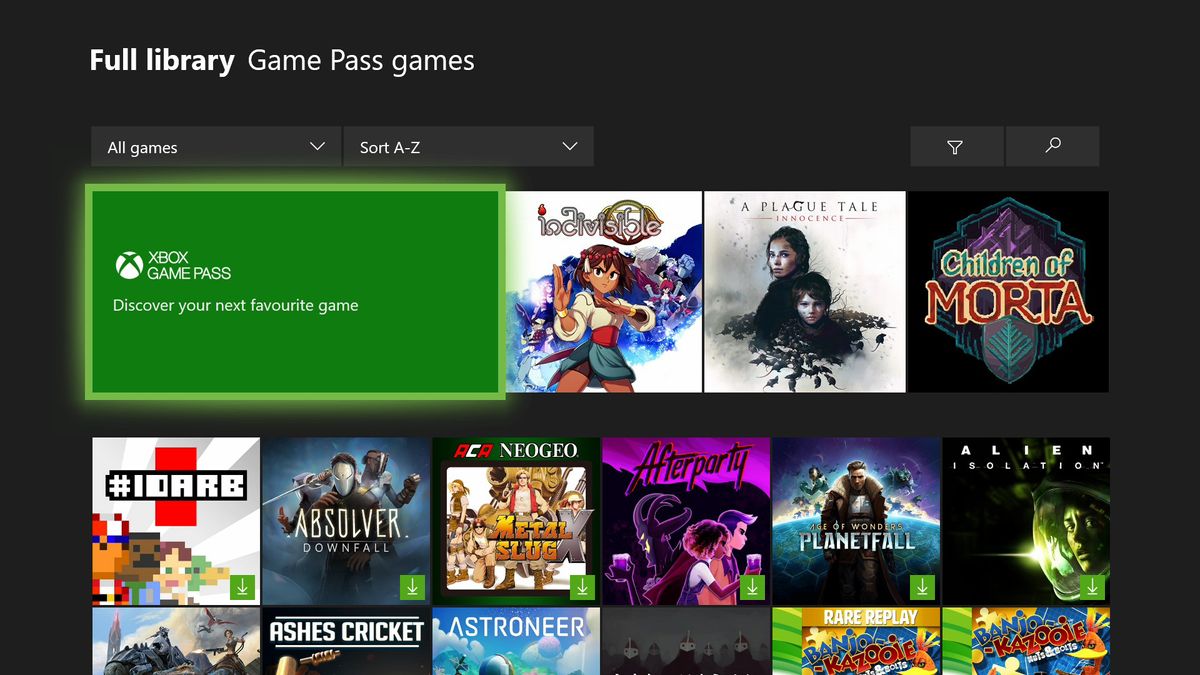The image displays the Xbox home screen, specifically showcasing the Game Pass section. The background is predominantly black, providing a stark contrast to the content. At the top of the screen, a bolded white font highlights "Full Library," next to which "Game Pass Games" is listed. Beneath these headings, there is a rectangular box with the label "All Games," accompanied by a drop-down arrow for sorting options, and another drop-down arrow positioned on the right side of this box. 

Below this, the text "Xbox Game Pass" is prominently highlighted in green. Adjacent to this section are images of various games, starting with "Indivisible." Following this, there are advertisements for "A Plague Tale: Innocence" and "Children of Morta," each accompanied by their respective logos. Additional game titles, including "Absolver: Downfall," "Neo-Geo Metal Slug," "Part Time UFO," "Planetfall," "Alien: Isolation," "Ashes Cricket," and selections from the "Rare Replay" collection, such as "Banjo-Kazooie," are also partially visible. Some game titles appear cut off, hinting at a broader selection beyond the visible screen area.